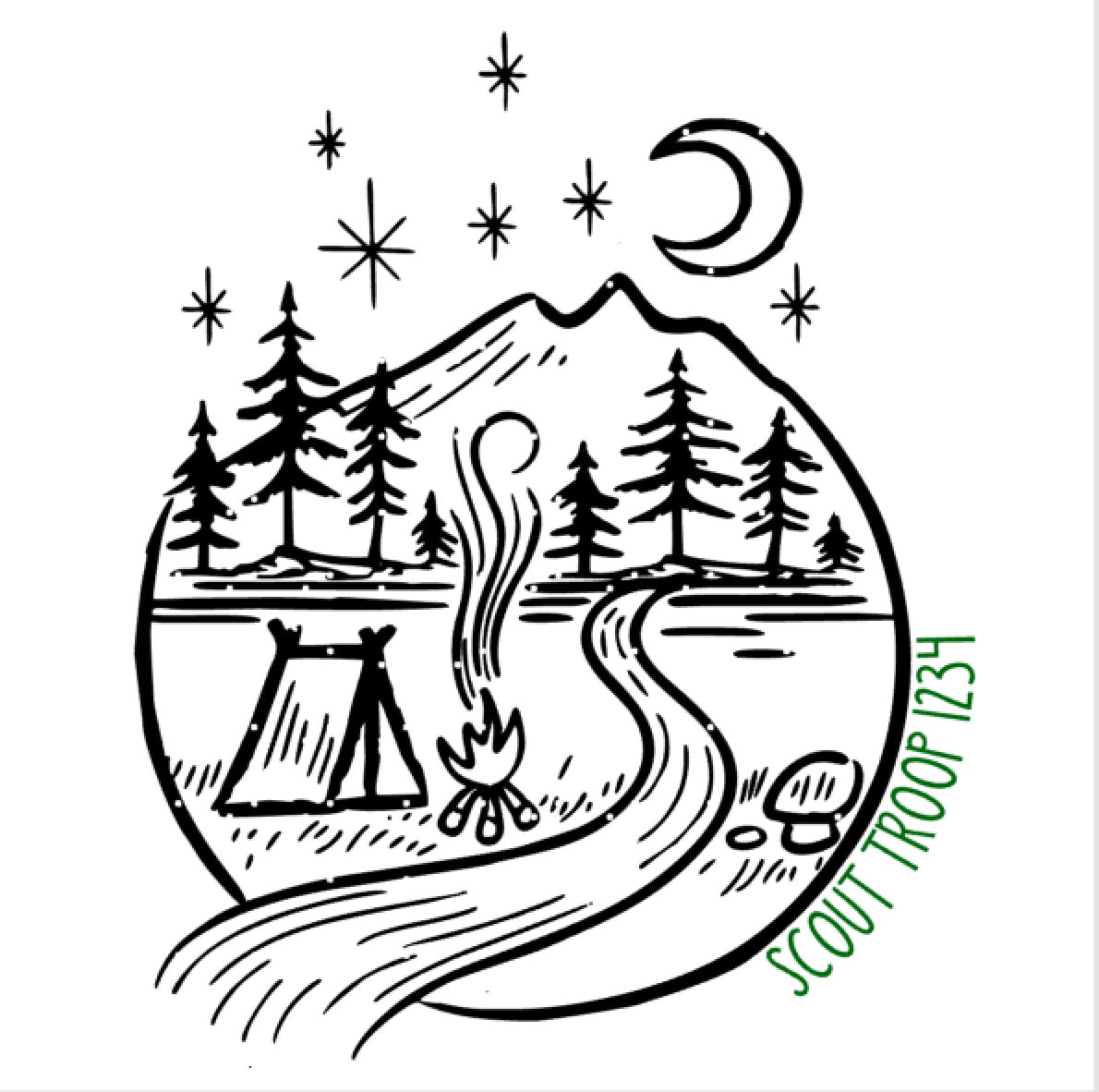The image depicts a detailed black and white drawing of a campsite scene, set within a circular frame against a white background. At the center of the frame, a flowing river or creek winds through the scene. To the left, there's a small tent with a campfire nearby, smoke rising up from the flames. On the right side of the circle, a mushroom can be seen. Tall trees, possibly pines, stand prominently in the background, suggesting a forest setting. Above the trees, the circle narrows into a peak, resembling a mountain, with stars scattered across the sky and a crescent moon on the right side. At the bottom right of the circle, in green text, the name "Scout Troop 1234" is inscribed. The entire illustration is rendered in black lines, highlighting the intricate details of the campsite scene.